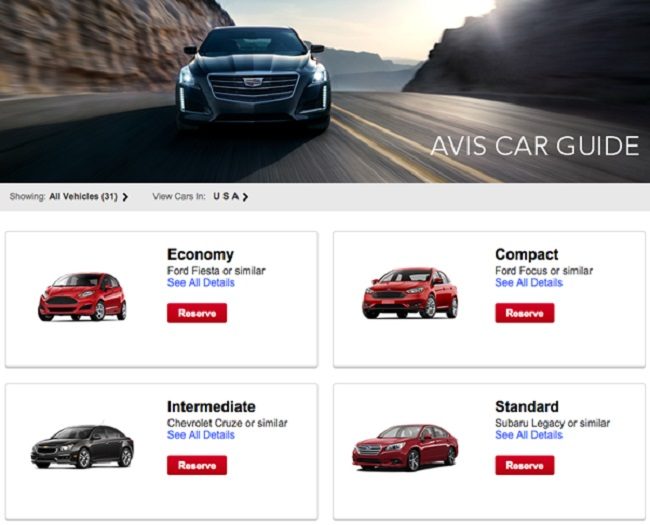The image serves as the cover for "Ava's Car Guide." At the top, there's a striking photograph of a black car driving towards the viewer on a highway with yellow lines. The highway is flanked by cliffs, with the early morning sun rising over the rocky terrain on the right side, casting a warm glow. Hills can be seen in the distant background. The words "Ava's Car Guide" are prominently displayed in the bottom-right corner of the photograph.

Beneath the main image, there's a subtitle that reads "Showing all vehicles 31." Under this, another line states "View all cars USA."

Below the text, there are four individual white-background cards displaying different car categories and their details:

1. **Economy**: On the left, with a red Ford Fiesta or a similar vehicle. There's a blue link that says "See all details" and a red button labeled "Reserve."
2. **Compact**: Positioned to the right, featuring a red Ford Focus or a similar model. This card also includes a blue "See all details" link and a red "Reserve" button.
3. **Intermediate**: On the bottom left, showing a black Chevrolet Cruze or a similar car. It includes the same blue "See all details" link and a red "Reserve" button.
4. **Standard**: Located at the bottom right, displaying a red Subaru Legacy or a similar vehicle with the blue "See all details" link and a red "Reserve" button.

The dominant colors in the image and text are red, blue, black, gray, white, and yellow, creating a visually appealing and informative guide.